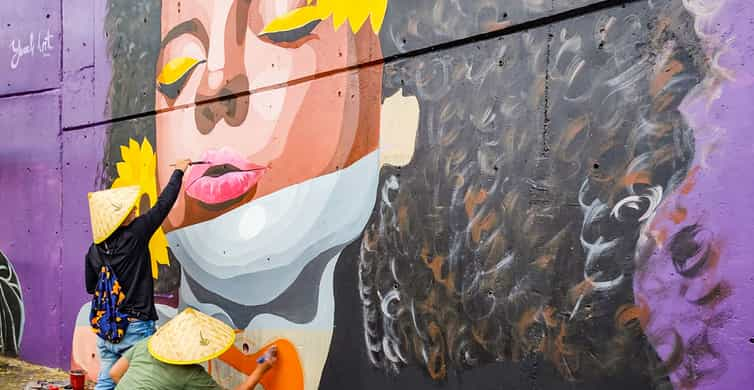In this vibrant outdoor scene, two artists are diligently painting a mural on a cement wall with a vivid purple background. The mural portrays a dark-skinned woman with her eyes closed, adorned with bright yellow eyeshadow and a bold eyeliner. Her pink lips are being carefully painted by one of the artists standing to the left, who is wearing a black long-sleeved shirt, blue jeans, a backpack, and a cone-shaped woven straw hat. This artist has a paintbrush in hand and appears to be methodically detailing the lips.

Meanwhile, another artist in a green short-sleeved shirt, also donning a similar hat, is kneeling and painting the lower portion of the mural. The mural's subject is depicted with large, luscious curly black hair streaked with burnt orange, gray, and white strands cascading down around her shoulders. She wears a white turtleneck pulled up over her chin, layered beneath a black sweater. The face of the mural presents a comic book-like, sultry expression, enhancing the mural's artistic depth and character. Additionally, a yellow flower decorates her hair, contributing to the mural's intricate and colorful design.